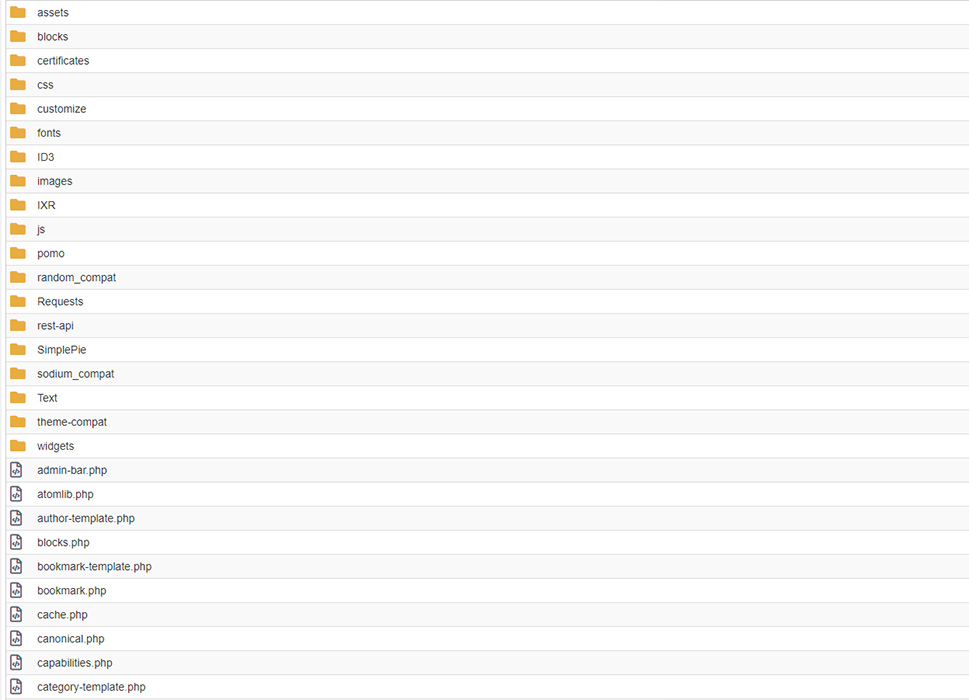The image depicts a computer screen displaying a detailed directory of files and folders. The screen is organized with horizontal lines alternating between white and gray, enhancing readability. Starting from the top left, there is a series of yellow folders labeled as follows: "assets," "blocks," "certificates," "CSS," "customize," "fonts," "ID3," "images," "IXR," "JS," "POMO," "random_compat," "requests," "REST-API," "SimplePy," "sodium_compat," "text," "themes-compat," and "widgets." 

Following the folders, there are several files with a rectangular icon, indicating they are PHP files. These include: "admin.php," "atom.php," "author-template.php," "blocks.php," "bookmark-template.php," "cache.php," "canonical.php," "capabilities.php," and "category-template.php." The meticulous organization of these directories and files suggests a structured and well-managed file system, likely used for web development or software projects.